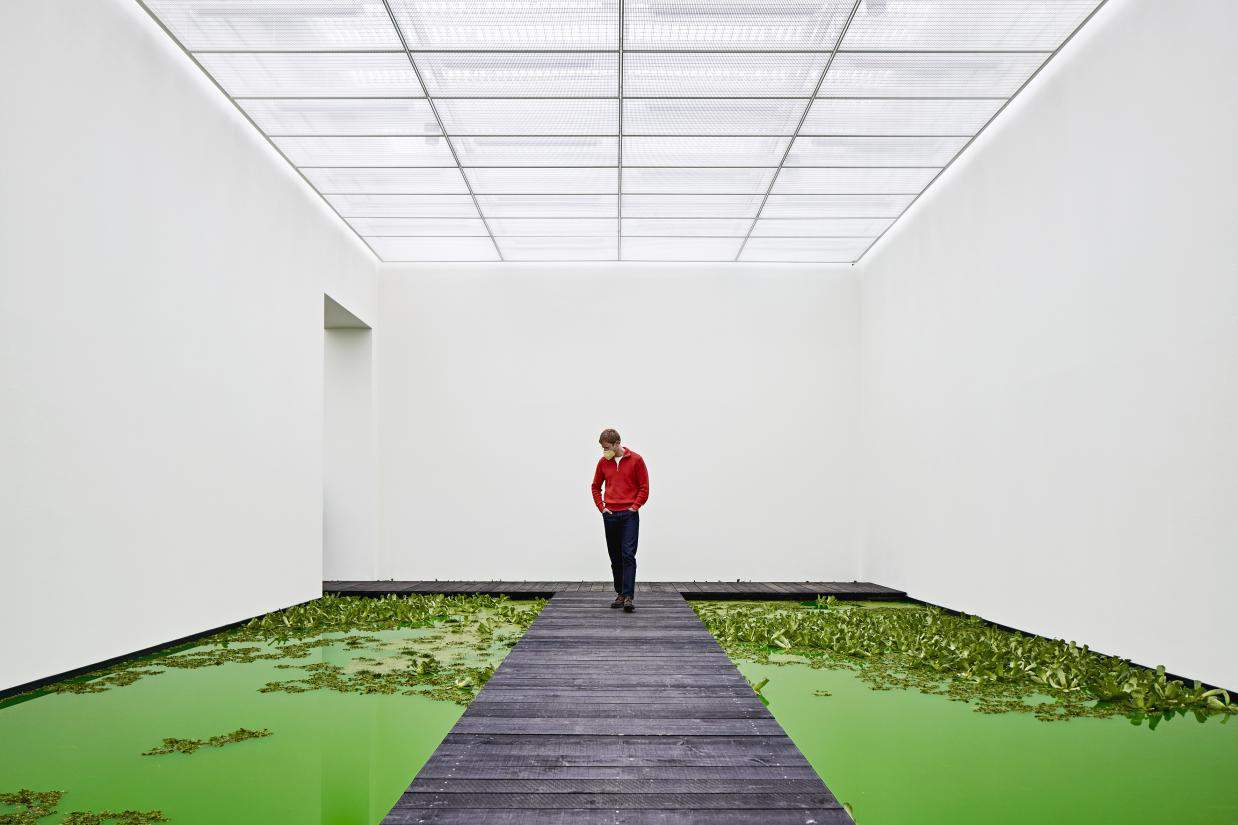In this captivating indoor photograph, a man is standing on a T-shaped wooden deck within a pristine white-walled room. The deck, which resembles a boardwalk or dock, is surrounded by striking lime green water and lush green plants that appear to be either growing in or floating on the liquid. The room is illuminated by soft white lights emanating from square panels on the ceiling. The man, with light brown hair, is examining the exhibit. He is wearing a red quarter-zip crew neck jacket over a white t-shirt, black pants, and a white face mask. His choice of attire complements the serene and primarily monochromatic environment, with the exception of the vibrant greens of the water and plants. The overall ambiance suggests a museum setting, inviting viewers to ponder the interaction between the deck's man-made structure and the natural elements of the exhibit.